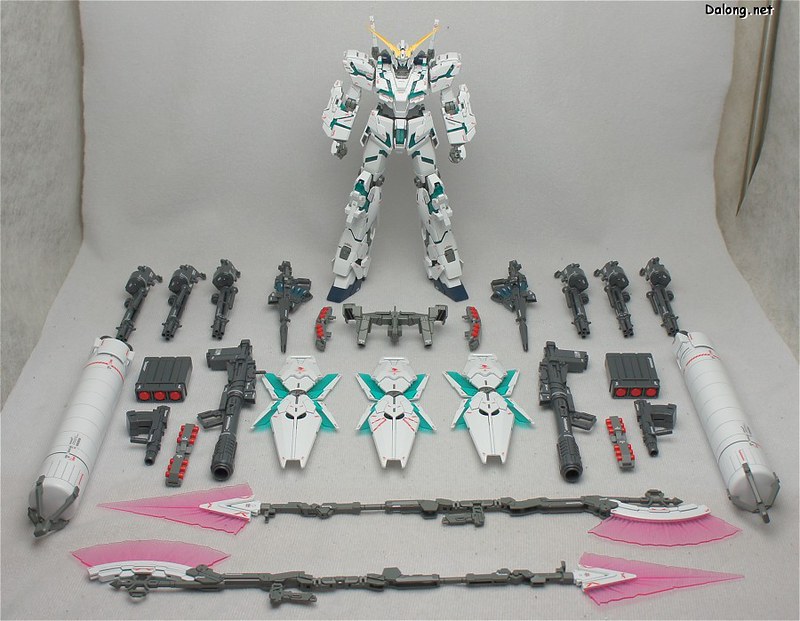This image showcases a detailed Gundam-style action figure, prominently positioned against a white, slightly bent background paper. The central toy is primarily white and teal, with accents of gray, black, and yellow. Noteworthy are its big, bulky arms and legs, and a small head adorned with two bright yellow antenna spikes. The symmetrical figure features an array of weaponry: four guns on each side, a center-mounted weapon, and additional accessories. Among these accessories are red and gray attachments near the feet, and sizable white cylindrical projectiles with red and gray details, positioned at both far ends of the image. At the bottom, two spear-like weapons with gray handles and translucent pink blades are visible. The image has a watermark in the top right corner reading "dalong.net," contributing to the well-organized, symmetrical layout.